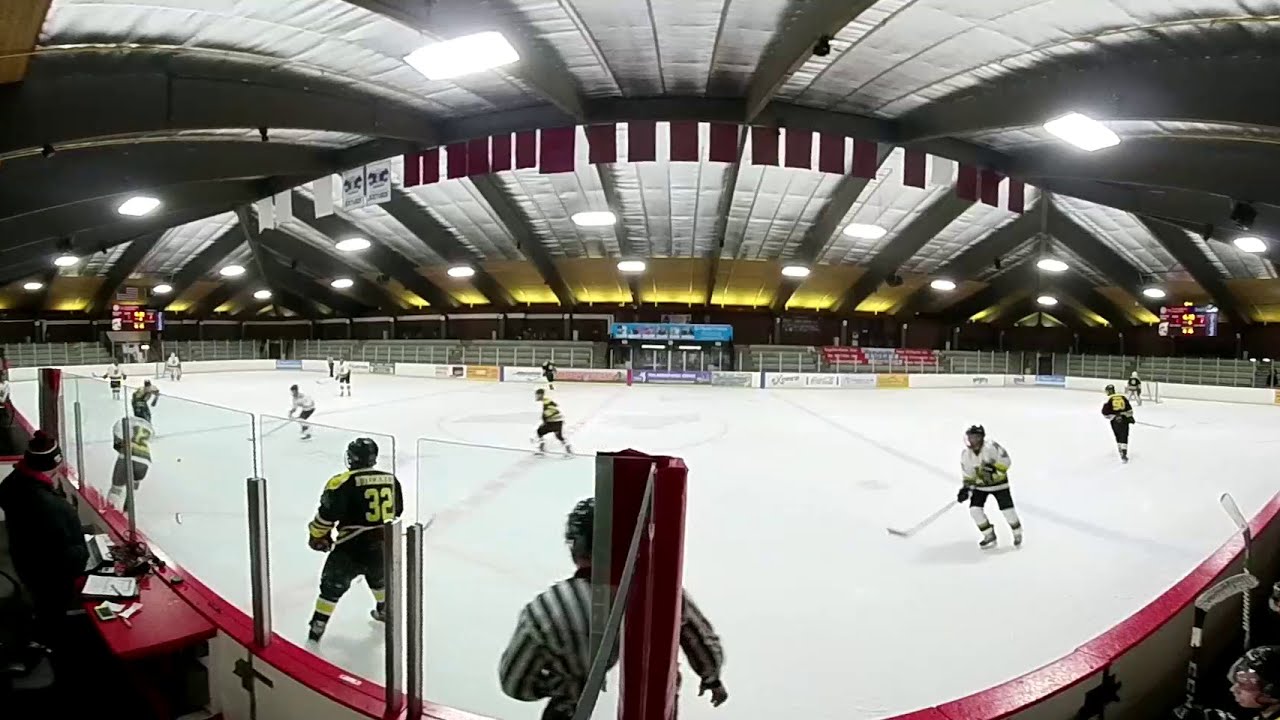This panoramic image captures the vibrant action of a hockey game on a large, light white ice rink. The rink appears slightly curved due to the wide rectangular panoramic view taken from the long side. Players in contrasting uniforms are actively engaged in the game; some are clad in black shirts with black pants and yellow accents, while others wear white jerseys, black pants, and white socks. Notably, player number 32, in black and yellow, stands on the left side, with player number 12 positioned just in front of him. Central to the image, a referee, identifiable by his black-and-white striped shirt, has his back to the camera.

The rink is bordered by a transparent barrier with a red top and white bottom, evident particularly on the left side where a person is seated at a desk with a red surface and white papers. The far-right corner features hockey sticks angled towards the ice and the side. Suspended above the rink, the ceiling, in a silver metallic hue, is adorned with numerous bright white rectangular lights and a series of banners—predominantly red, with a few white ones on the left—hanging down. The scene is set indoors during an active game, and the ambiance is illuminated by downward-facing lights casting an evenly distributed white glow over the ice.